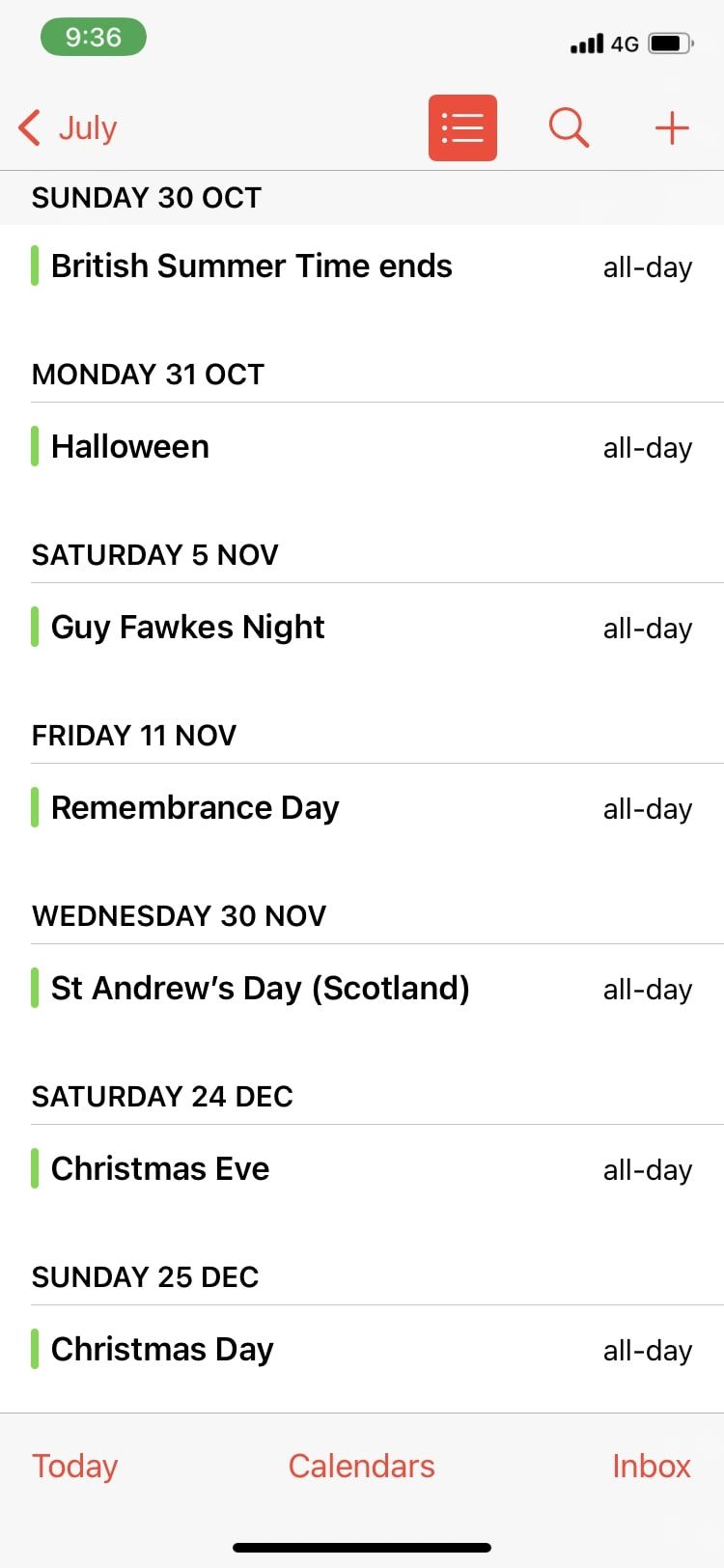The image showcases a planner app displayed on a smartphone, open to the month of July. The month's name, "July," is prominently written in red at the top left of the screen, and to the right, there are icons for navigating back, listing items, searching, and adding entries, all depicted in red. Below the month title, events are listed by date:

- On Sunday, 30th October, "British Summer Time Ends," marked as an all-day event.
- On Monday, 31st October, "Halloween," which also spans the entire day.
- On Saturday, 5th November, "Guy Fawkes Night/Day."
- On Friday, 11th November, "Remembrance Day," another all-day event.
- On Wednesday, 30th November, "St. Andrew's Day" in Scotland, marked for the whole day.
- On Saturday, 24th December, "Christmas Eve."
- On Sunday, 25th December, "Christmas Day," both noted as all-day events.

Each event on the planner has a green line on the left side. At the bottom of the screen are navigation tabs: "Today" on the bottom left, "Calendar" at the bottom center, and "Inbox" on the bottom right.